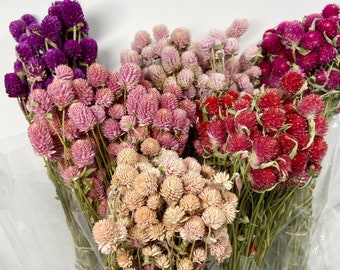This photograph captures six bouquets of vibrant flowers, each intricately wrapped in translucent plastic and artistically arranged against a white, slightly grayish background. The bouquets are aligned in a V shape, central to the image. Starting from the center, the largest bundle features cream-colored, oval-shaped flowers reminiscent of cotton candy balls. To the left, there are clusters of vivid purple and soft pink flowers, while the right side showcases bouquets of deep red and strawberry-pink blooms. Interspersed among the blooms, long, light green stems and grass-like greenery add a natural touch, enhancing the overall arrangement. The stems are subtly visible, emphasizing the delicate yet structured composition of the display. The entire array presents a harmonious blend of colors and shapes, creating a visually striking and detailed floral ensemble.